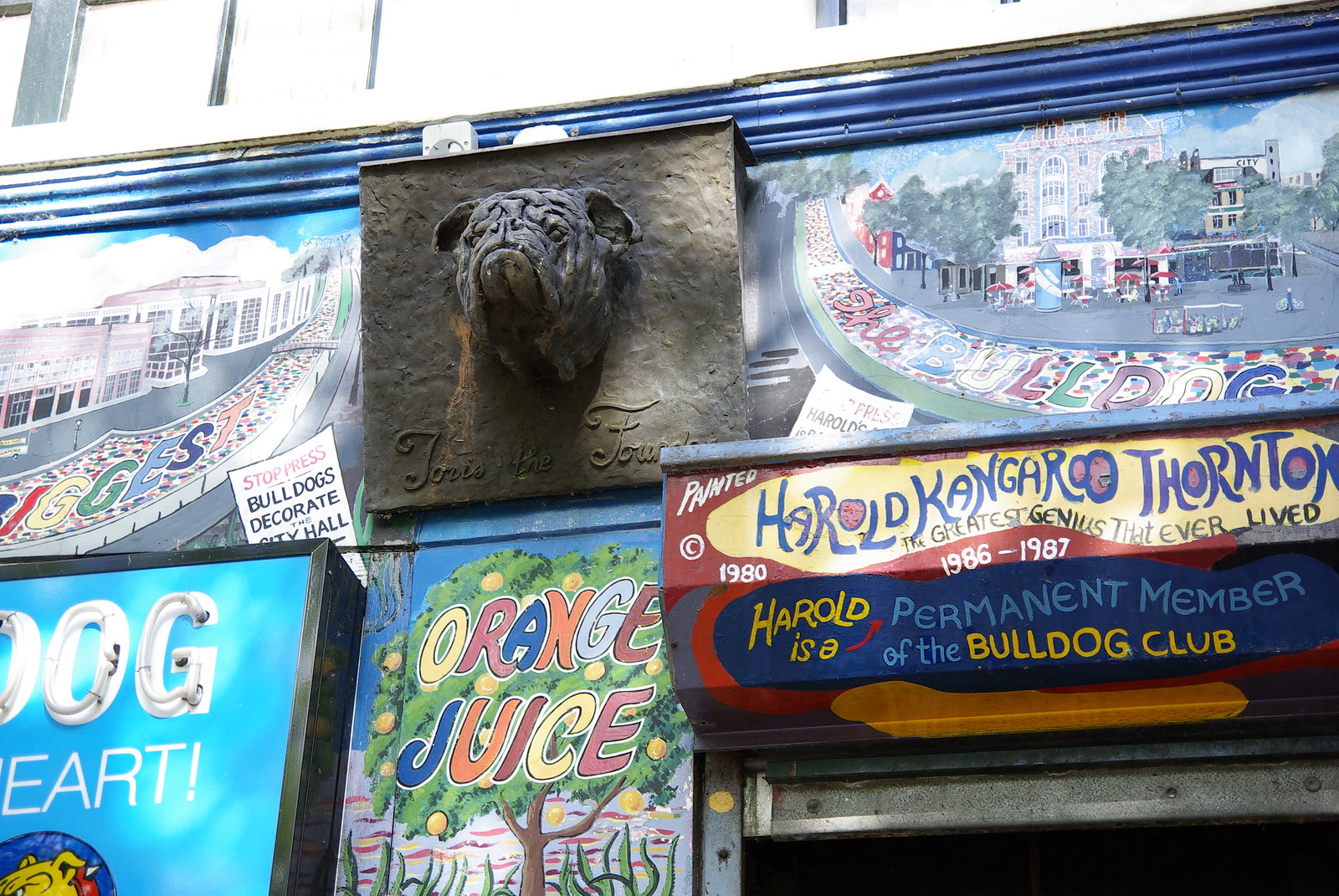This detailed image captures the lower front facade of a building on a bright, sunny day. The central focus is an intricately detailed brass plaque featuring a cast bronze bulldog bust, slightly projecting out with a dark grayish-brown hue. Below the bulldog, an inscription in cursive is partially obscured and difficult to read.

The plaque is flanked by colorful painted murals on both sides, depicting various scenes and events. On the left side, an eye-catching painting showcases a vibrant building front with a banner proclaiming, "Stop the presses, bulldogs decorate the city hall." This message complements the central bulldog theme.

To the right of the bulldog, another vibrant mural displays an elongated building facade featuring the word "BULLDOG" prominently. Below these murals, the lower row continues the narrative. Directly beneath the bulldog, a lively painted image of an orange tree is captioned with the words "ORANGE JUICE" in multicolored, cursive text. To the far right, an awning with striking, bright colors marks another painted segment that reads, "Harold Kangaroo Thornton, 1986 to 1987, the greatest genius that ever lived," all set against a blue backdrop. It also notes, "Harold is a permanent member of the Bulldog Club," with "Harold" and "bulldog" in yellow, and the other text in blue.

Additionally, a neon sign displaying the word "DOG" in lit letters can be seen adorning the left side towards the lower row, further enhancing the playful and thematic visuals of this captivating building facade.